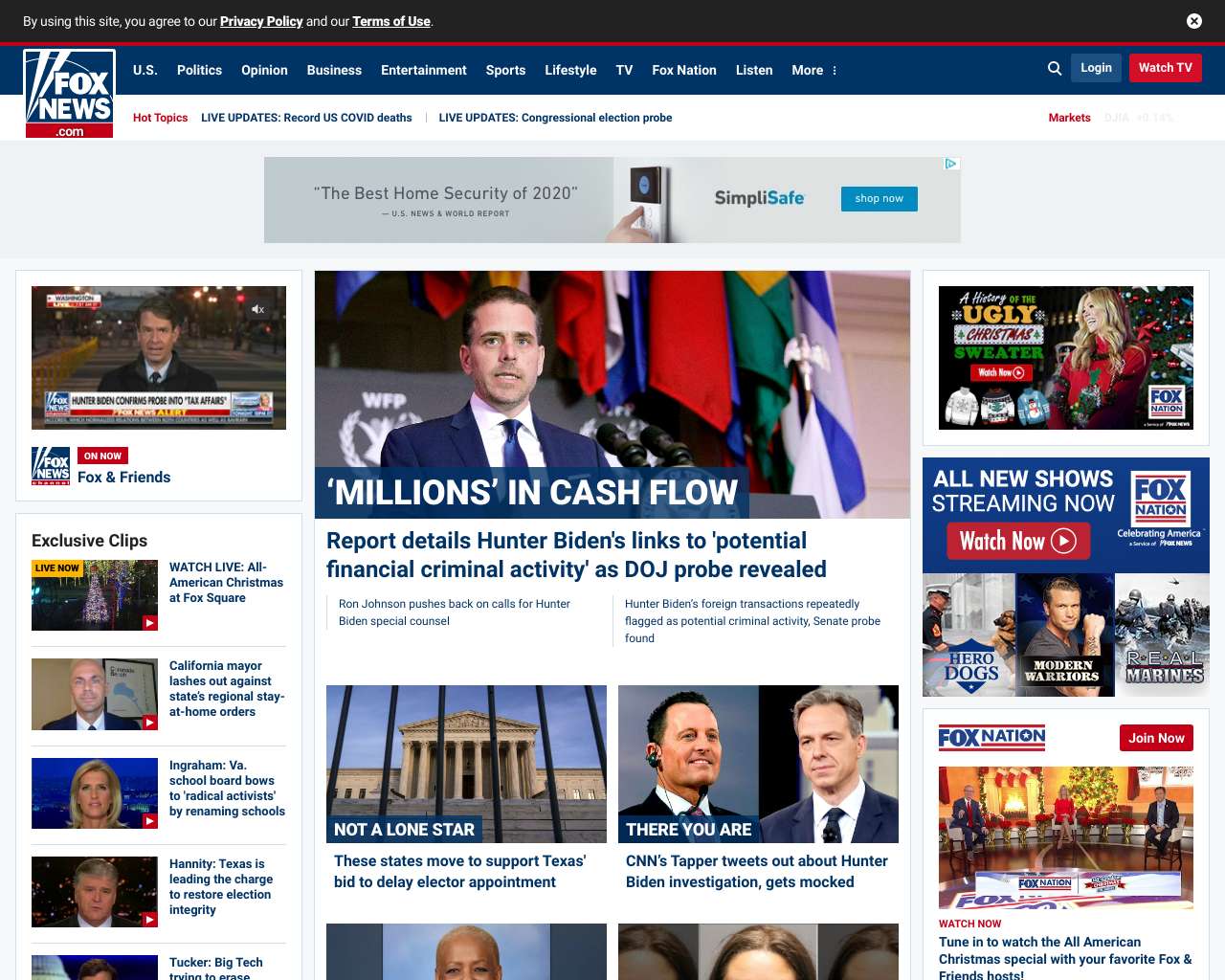The image depicts the Fox News website interface. The majority of the page features a clean, white background. At the very top, a black banner bar displays a message in white text: "By using this site you agree to," followed by bold, white text reading "Privacy Policy" and "Terms of Use." To the far right of this banner, there is a white circle with a black 'X' inside it.

Directly below this black banner, the FoxNews.com logo is prominently displayed along with a thin red line. Following this, a blue banner bar spans the width of the page. This blue bar contains navigation options listed in white font: "U.S.," "Politics," "Opinion," "Business," "Entertainment," "Sports," "Lifestyle," "TV," "Fox Nation," "Listen," and a "More" option indicated by three dots. Additionally, there is a white magnifying glass icon positioned for search functionality.

To the right of these navigation options, there is a light blue button with white text that reads "Log In," alongside a red button with white text that reads "Watch TV."

Below the blue banner bar, a white banner bar features "Hot Topics" in red font, followed by two lines of blue text: "Live Updates: Record U.S. COVID Deaths" and "Live Updates: Congressional Election Probe," indicating current and important news highlights.